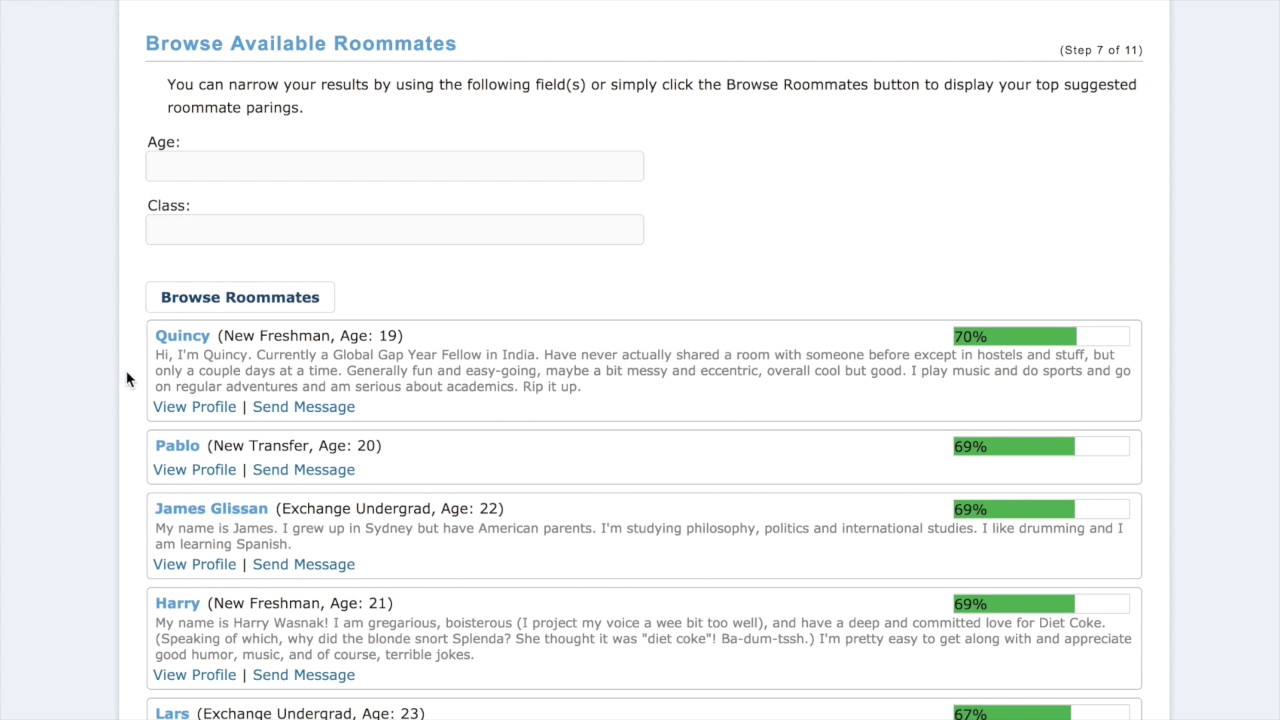The image showcases a digital interface designed for browsing available roommates. The layout consists of two grey panels flanking a central screen. At the top of this screen, the title "Browse Available Roommates" is prominently displayed in blue.

Below the title, there are input fields where users can enter specific preferences such as age and class to filter potential roommates. Further down, a list of roommate profiles is displayed. Each profile provides a brief introduction, highlighting personal details and interests. For example, one profile reads:

_"Hi, I'm Quincy, currently a Global Gap Year Fellow in India. I've never actually shared a room with someone before except in hostels and stuff, but only for a couple of days at a time. Generally fun and easygoing, maybe a bit messy and eccentric. Overall, cool but good. I play music, do sports, and go on regular adventures, and I'm serious about academics."_

Each profile includes a "View Profile" link for more detailed information and a "Send Message" link for direct interaction. Additionally, each roommate has a compatibility score displayed on the right-hand side, ranging from 67 to 70 for the profiles shown.